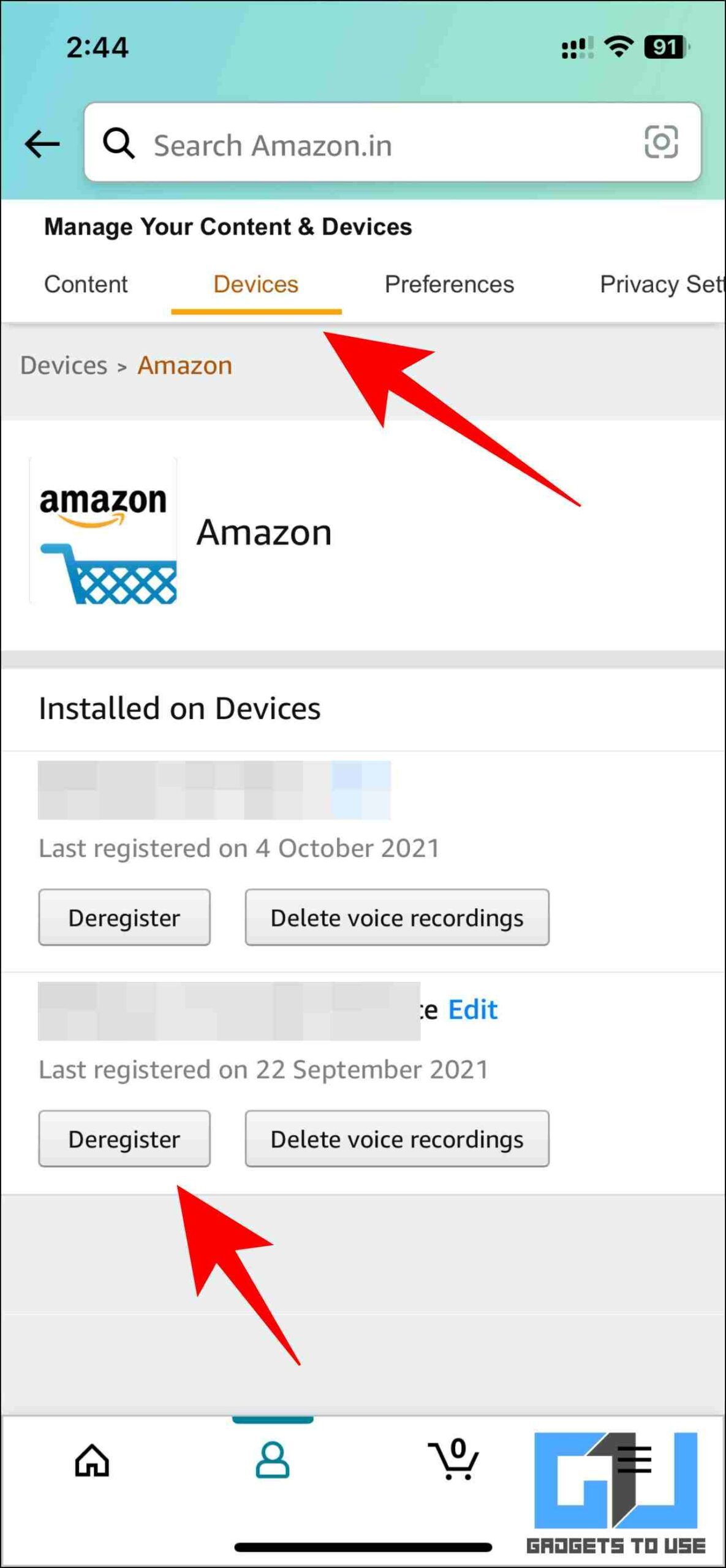This is a detailed descriptive caption for the provided voice caption:

---

Screenshot of an Amazon.in page displaying the 'Manage Your Content and Devices' section. The page features the Amazon logo with a shopping cart icon prominently at the top. The toolbar is highlighted with a turquoise strip across the top, approximately three to four inches wide, which adds a decorative touch to the otherwise simplistic grayscale interface.

In the main content area, there is a list of devices, noting one that was last registered on October 4th, 2021. Directly below each device listing, there are options to 'Deregister' or 'Delete Voice Recordings,' with a large, bright red arrow emphasizing the 'Deregister' button. The arrow is particularly eye-catching, guiding the viewer's attention to this option clearly.

The Amazon shopping basket icon, located near the top, is dark blue and stands out against the neutral tones of the rest of the page. At the bottom of the page, there is some partially obscured or unclear text, possibly including the word "groggets," although its exact meaning or context is uncertain.

Overall, the page’s layout is straightforward, with functional design elements highlighted subtly for user navigation.